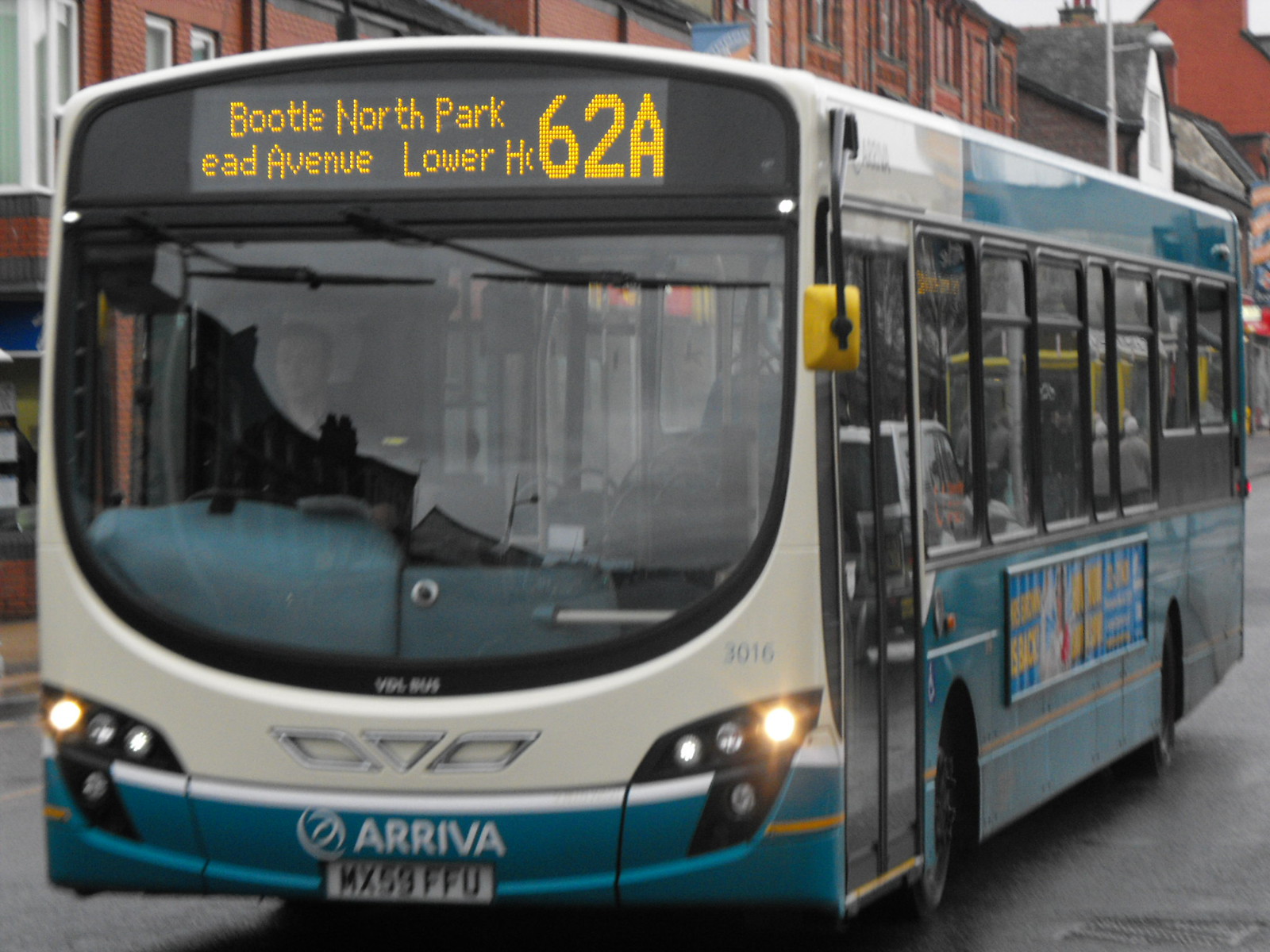This image features a bustling downtown city scene in the middle of the day. Dominating the center is a large blue and white passenger bus with a license plate reading MX-59FFU. The bus is in motion, navigating a paved asphalt road. A sign on the front of the bus indicates its route, which includes Boodle North Park, Ede Avenue, Lower 62A. The driver is positioned on the right-hand side, adhering to local driving norms. The bus, adorned with blue trim along the bottom, displays the word "Arriva." There is also an advertisement along the lower side of the bus. To the left of the bus, a sidewalk lined with various buildings adds to the urban atmosphere. Visible colors in the scene include shades of gray, blue, orange, yellow, black, and brown, enhancing the vibrant city setting.